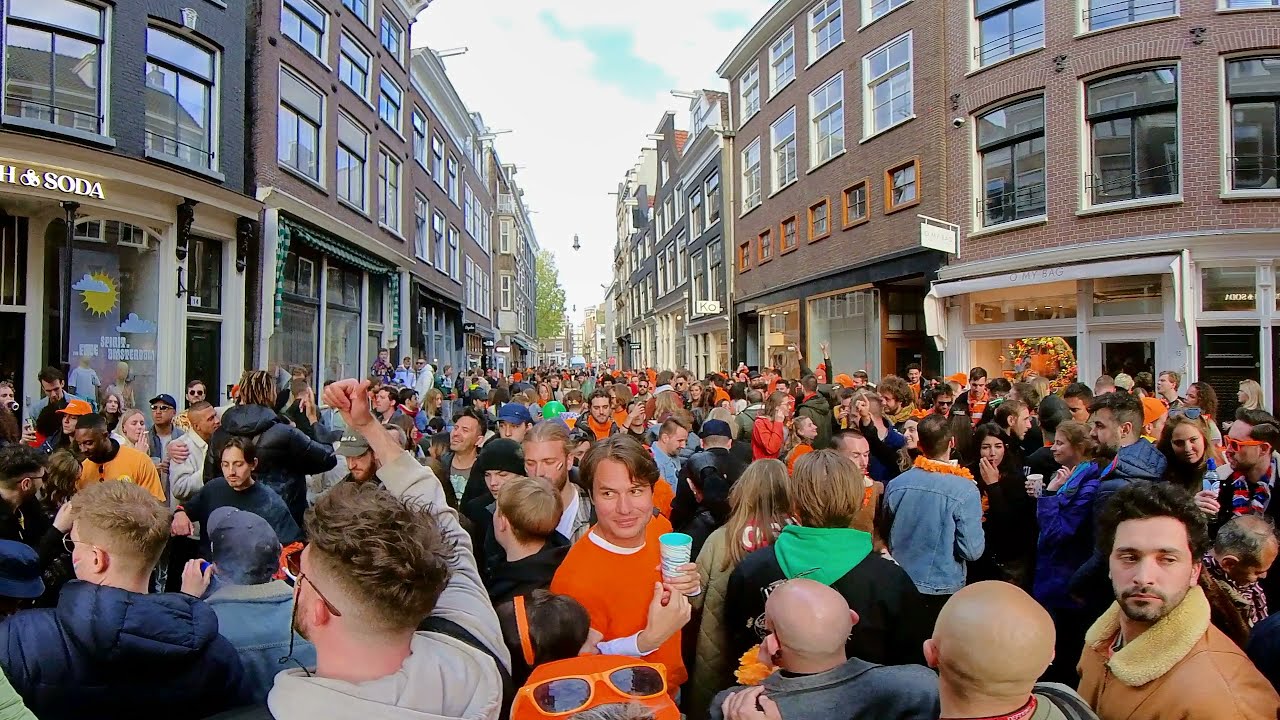The image depicts a bustling, crowded pedestrian street during what appears to be a fall celebration. The sky is a light blue, dotted with large white clouds. The street is flanked by multi-storied town row houses, predominantly made of reddish-brown brick, each adorned with numerous windows. At street level, the buildings feature various commercial storefronts, including one partially visible sign that reads "Ann's Soda" and another sign with the letters "KO," suggesting an upscale shopping area. 

A significant number of the crowd participants, comprising young men and women, are dressed in orange attire—shirts, sunglasses, leis—indicating a possible theme or festivity such as Halloween. Among them, one individual is noted to be smoking while another wears a light brown jacket with a white fur collar. The dense crowd of people holds cups and appears celebratory, integrating into the street so thoroughly that the pavement itself is obscured. In the background, beyond the sea of people, several trees are visible, contributing to the area's vibrant ambiance.